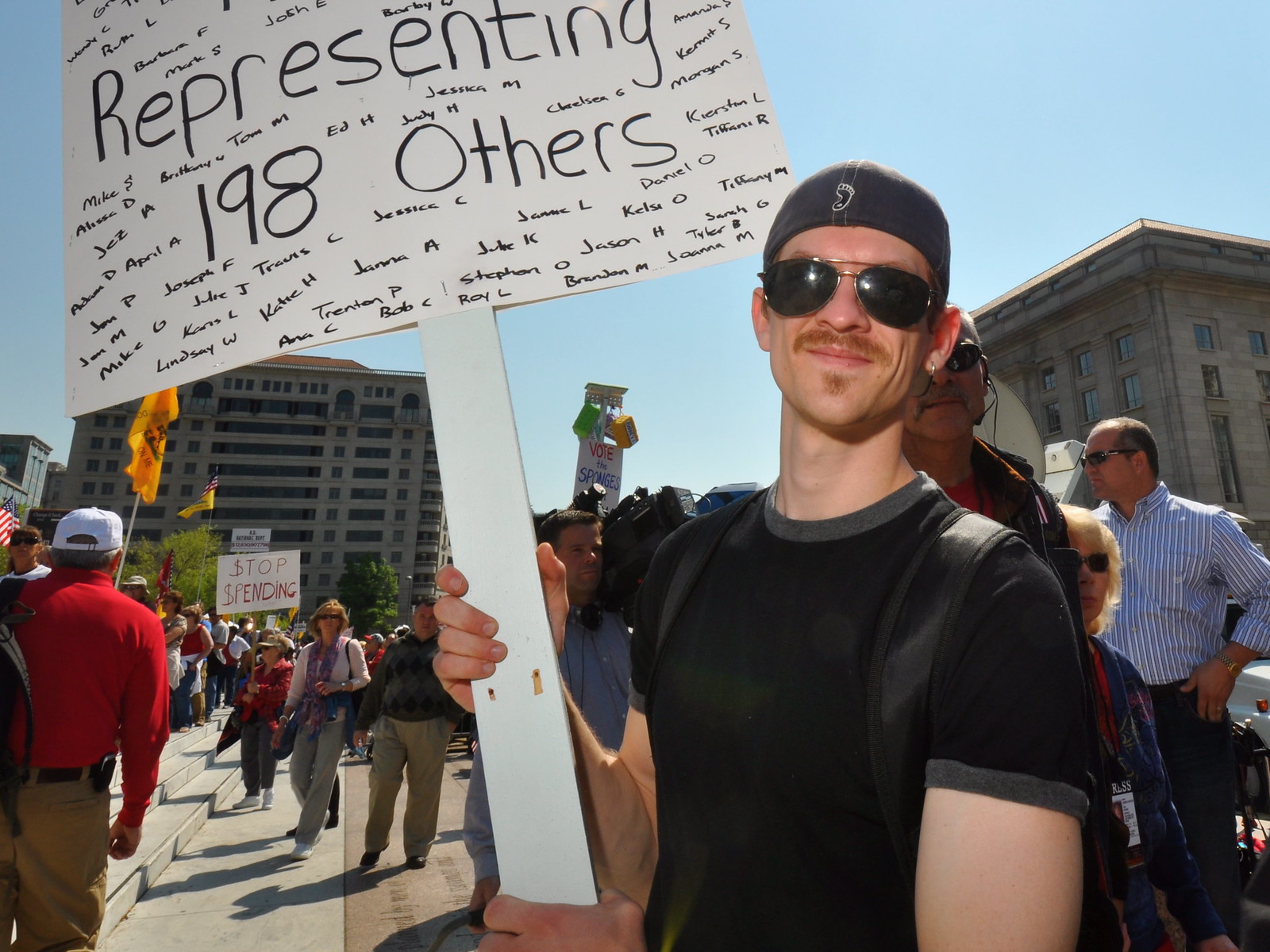In the photograph, a protest unfolds in an outdoor square bordered by concrete buildings, likely near a courthouse or civic structure. At the center of the image stands a man dressed in a black t-shirt with gray trim, black sunglasses, and a backward black cap. He firmly grasps a white sign on a wooden post with both hands. The sign bears the message "Representing 198 others" in black marker, surrounded by a multitude of handwritten first names like Jessica, Kelsey, Jason, Jean, Tiffany, Ken, Trenton, Katie, and Lindsay, indicating those he represents. The spacious stone or concrete walkway teems with protesters, some holding signs. To the left, a woman hoists a red-lettered sign reading "Stop Spending." The scene is lively, suggesting a mid-day rally with a crowd that fills the center of the image. The atmosphere is charged with activism, underscoring the participants' call for government action on spending and representation.